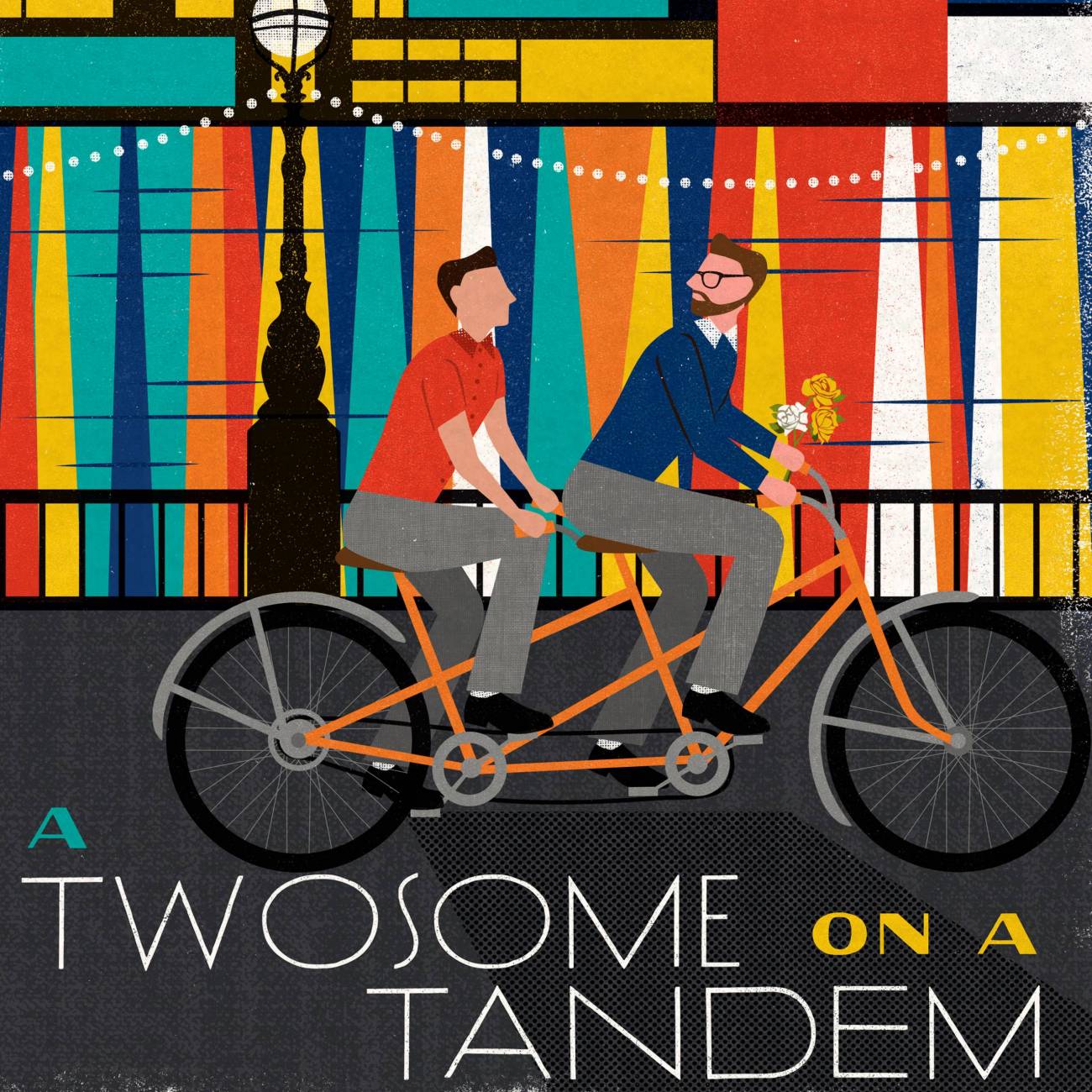A vibrant and whimsical art piece, this tall, square illustration features two men riding a tandem bicycle. The man in the front seat is Caucasian with brown hair, a brown beard, and a mustache. He is dressed in a blue shirt and gray pants, holding a trio of flowers—two orange and one white. The man seated at the back is also Caucasian, sporting black hair and an orange short-sleeve shirt, paired with gray pants and black shoes. The light orange bicycle they ride glides over a paved surface. 

Above them, a string of lights is suspended, originating from a lit black lamppost. The background is a mesmerizing multicolor tie-dye of blues, yellows, whites, and oranges, adding a magical atmosphere to the scene. Behind the riders is a wall and a blackish gate, enhancing the urban aesthetics of the composition.

The caption within the image reads "A" in an aquamarine hue, followed by "twosome" in a white city-style font, the number "1A" in yellow, and finishing with "tandem" again in a white city-style font.